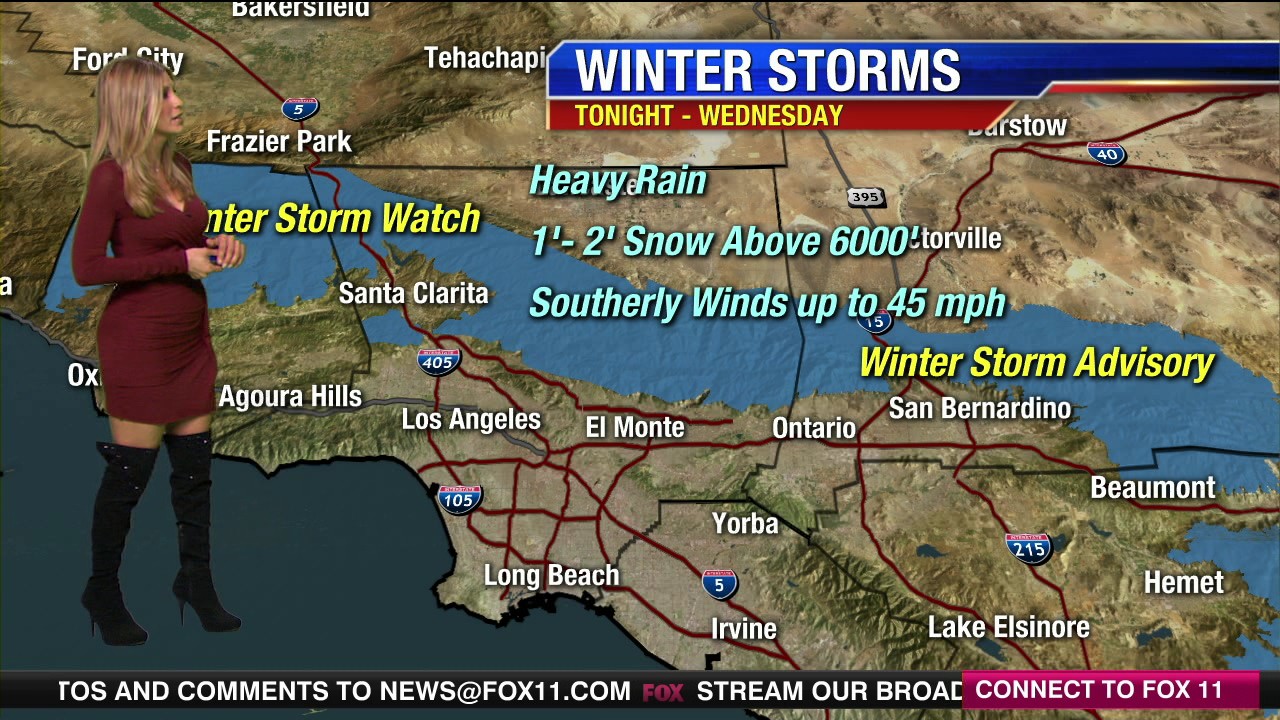This horizontal screenshot captures a local Los Angeles weather broadcast. A female meteorologist, standing on the left side of the image, is presenting in front of a topographical map of Southern California. She’s wearing a chic, long sleeve maroon dress paired with high stiletto black boots, and her long dark blonde hair is left flowing. The entire map background highlights the region’s detailed topography, including Los Angeles and Long Beach neighborhoods, and vivid color codes indicating weather alerts.

At the top right corner of the screen, a blue stripe with white letters announces, "Winter storms tonight through Wednesday," followed by specifics in yellow text. The details inform viewers of a winter storm watch, advisory, and heavy rain in some areas. Notable weather conditions include 1-2 inches of snow above 6,000 feet and southerly winds up to 45 mph.

A black banner with white and pink text runs across the bottom, providing the web address 'news at fox11.com' and prompting viewers to stream the broadcast and connect with Fox 11. The meteorologist appears engaged, possibly discussing the winter storm's impact on the region's various neighborhoods and interstates, as evident from numerous labels on the map.